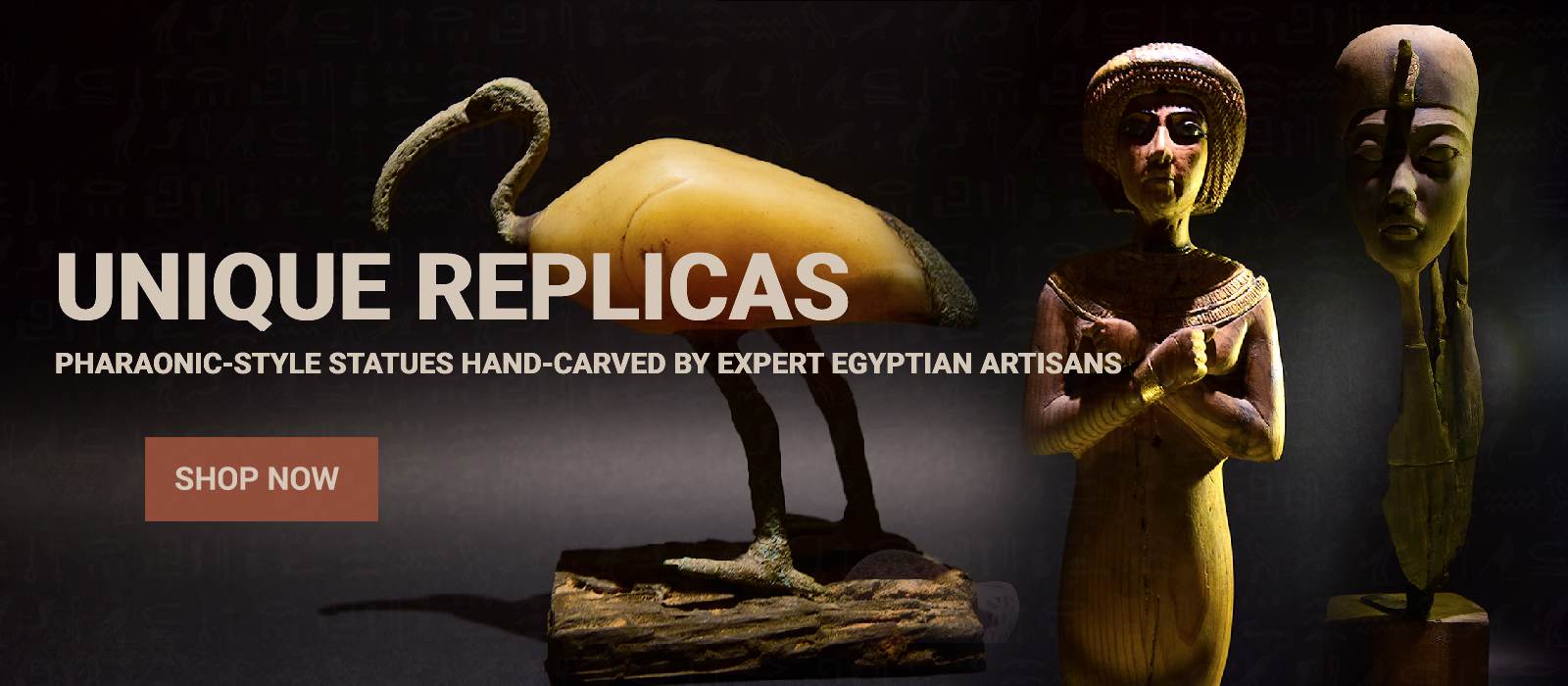This photograph displays a cropped web page focusing on exquisitely detailed, hand-carved, pharaonic-style statues crafted by expert Egyptian artisans. Against a deep, dark background, three prominent artifacts are showcased: one features a face resembling ancient Egyptian artwork with folded arms, another displays a face with intricate detailing, and the centerpiece is a bird with a beak reminiscent of a toucan, standing on what appears to be petrified wood or rock. Overlaying the images is text that reads "unique replicas, pharaonic-style statues hand-carved by expert Egyptian artisans," accompanied by a "shop now" button in the corner, suggesting these items are available for purchase.